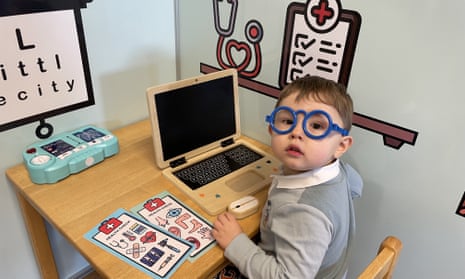In this image, a young boy, likely around four years old, sits at a wooden desk and chair setup. He is wearing large, round blue glasses and a gray shirt with a white collar. The boy appears to be in what looks like a play or learning environment, possibly themed to look like a doctor's office. In front of him is a toy or possibly real laptop that is open but powered off, accompanied by a computer mouse to his left. Beside his left hand are two study sheets adorned with various symbols, presumably representing the human senses. Behind him, there are illustrations on the wall including an eye chart with the words "Little City" on it, and a medical chart with check marks and a stethoscope. The background wall is white, and a blue object, though unclear what, is visible in the background. The boy, with mousy brown hair and a chubby face, is looking directly at the camera, creating a charming and detailed portrait of a young child engrossed in his imaginative environment.